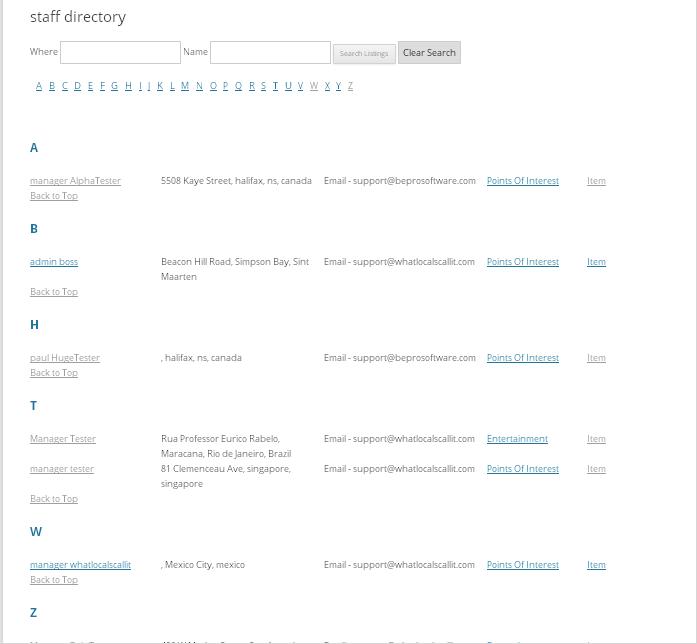The image features a white background with a gray border along the left, right, and bottom edges, forming a rectangular shape. In the top left corner, the text "Staff Directory" is prominently displayed. Below this heading, there are two text boxes labeled "Name" for users to input search criteria. Adjacent to these boxes is a gray button labeled "Clear Search."

The directory also includes a series of blue hyperlinks representing the letters A through Z for easy navigation. The remaining content is somewhat blurry, but certain details are discernible. For instance, under the letter "A," there is an entry for "Aloha Tester," listed with an address that starts with "55" and a location in Halifax, NS Camden. The contact email is partially legible as "support at [something]."

Similarly, under the letter "B," there is an entry for "Admin Boss," with an address that begins with "Beacon Hill" in Sampson Bay. The email contact reads "support at [something].com." Both entries include blue hyperlinks labeled "points of interest."